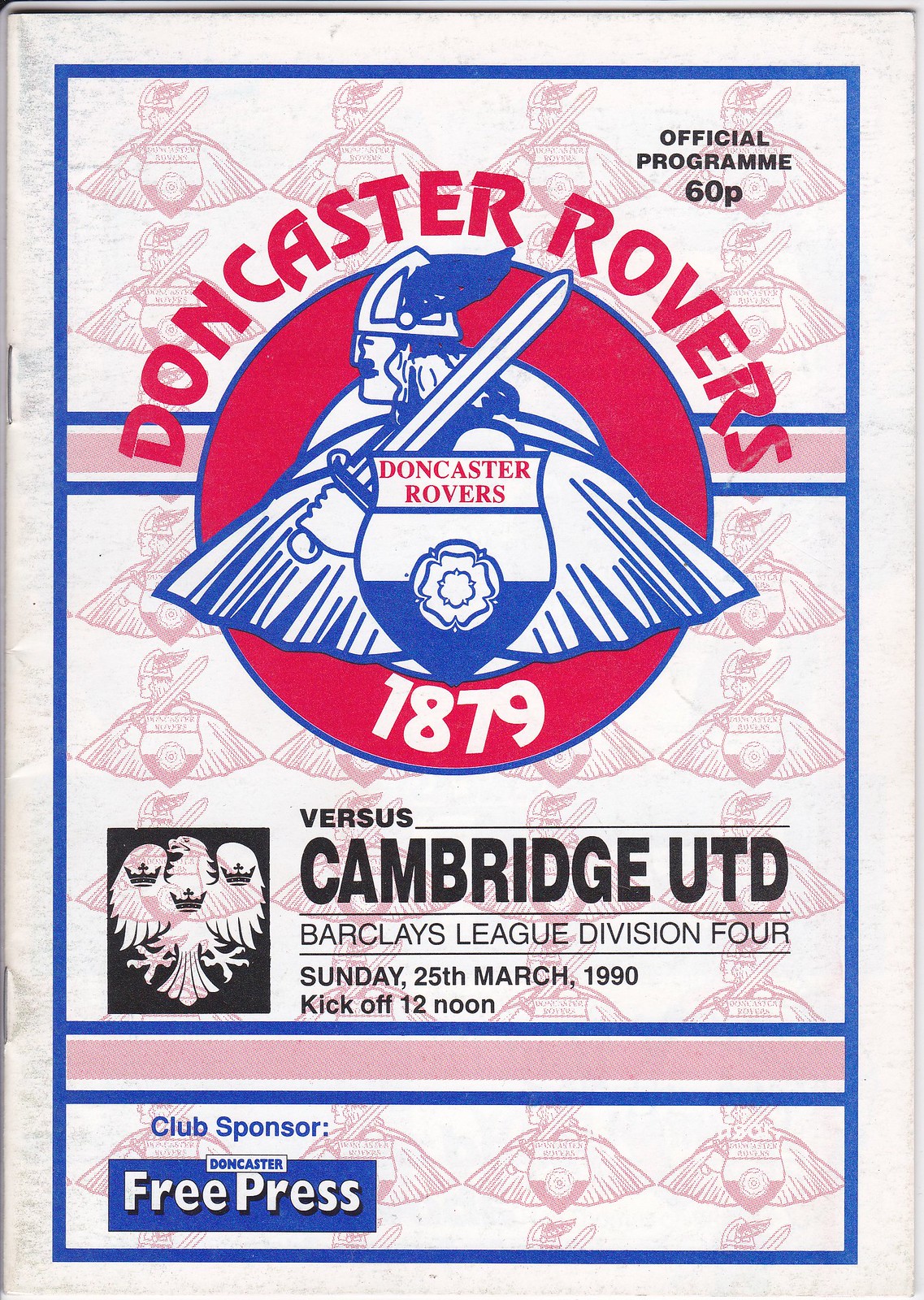The image is an official match program for Doncaster Rovers, featuring a predominantly white background with a blue border framing the page. The top right corner displays "Official Program" in black lettering. Below this, "Doncaster Rovers" is prominently written in red, along with the year "1879," which is the year the club was established. The program includes an image of a mascot that resembles a warrior adorned with a feathered helmet and holding a long sword. Below this, the text "versus Cambridge UTD" is written in black, indicating the opposing team for the match. The event details "Barclays League Division 4, Sunday 25th March 1990, Kick off at noon" are also present. At the bottom of the program, "club sponsor" is mentioned along with "Doncaster Free Press." The program has an aged appearance, giving it a vintage feel, possibly from a magazine or similar publication.